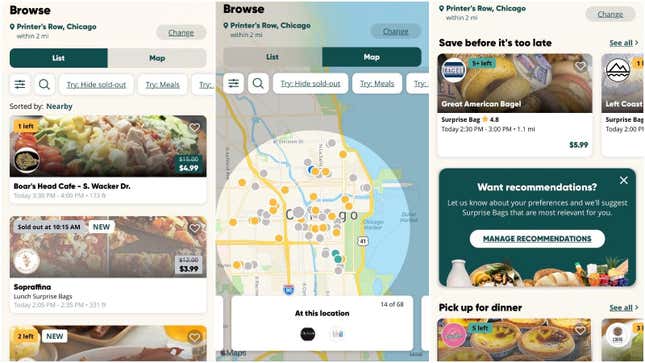This is a detailed screenshot showcasing a side-by-side comparison of nearby restaurants. On the left side of the screenshot, at the top, there's a header that says "Browse" in large text. Directly below that, in green text, it reads "Printer’s Row, Chicago," indicating the location being searched. Two rounded buttons are situated below this section. The left button, highlighted in green, is labeled "List," while the right button, in grey, is labeled "Map." Beneath these buttons, there are icons for filtering options including a filter icon, a search icon, an option for hiding sold-out items, and finally a "Try Meals" button.

Further down, the sorting method "Sorted by Nearby" is displayed, with "Nearby" emphasized in green. Under this sorting label, two restaurant listings are visible. The first restaurant is "Boar's Head Cafe," located on South Wacker Drive. The second restaurant listed is "Soprofina."

On the right side of the screenshot, a map is displayed, showing the same area with various circular pins indicating the locations of different restaurants. This map visualization provides a spatial representation of the eateries in the Printer’s Row, Chicago area.